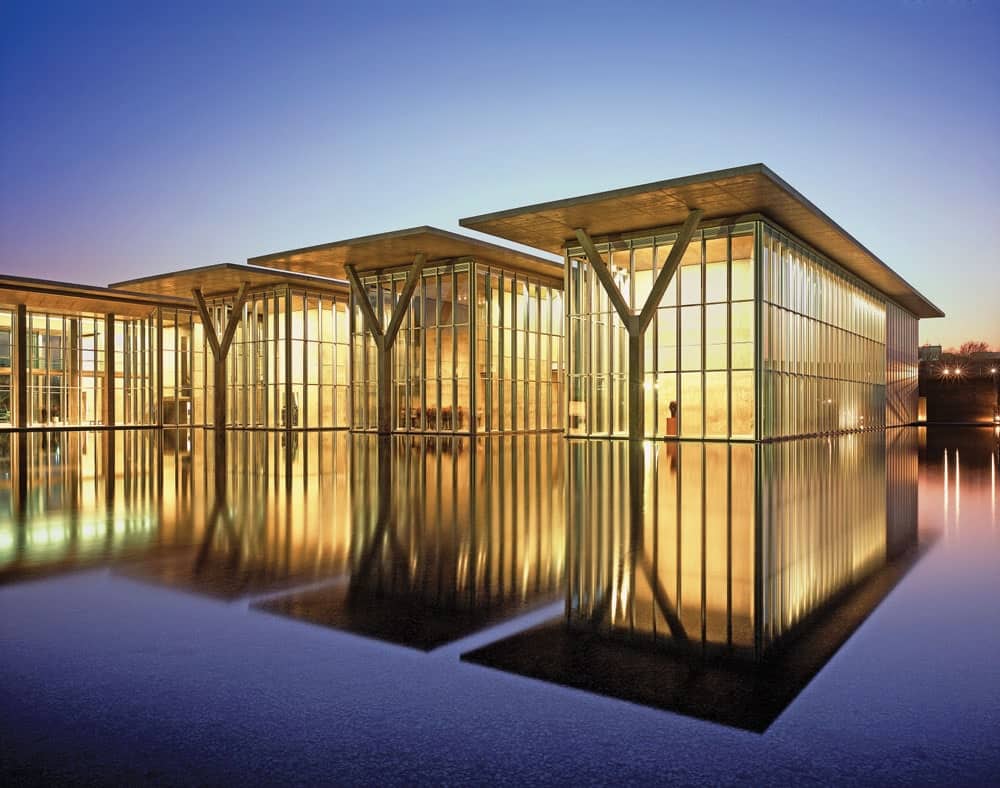The image depicts four small, storage shed-like structures arranged in a square formation. Each shed emits a bright, yellowish light, making them stand out against the scene. These illuminated sheds are set atop a deep blue body of water, which gives a reflective glow. It appears to be transitioning from evening to nighttime, as the scene is dimly lit but not entirely dark. The sheds seem to be accessible, with possible doors visible for entry. They rest on a black foundation that provides support and stability, enhancing the contrast with the vivid blue water below. The overall setting feels tranquil and almost surreal, with the sheds' warm glow contrasting the cool tones of the surrounding water and evening sky.